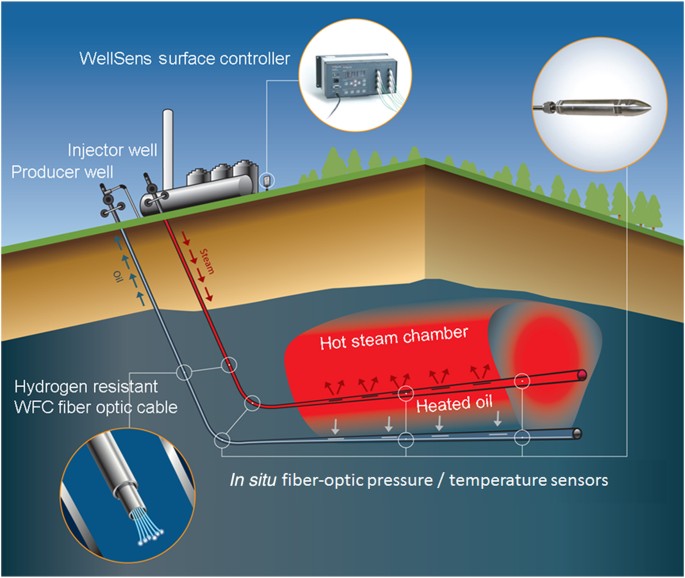The image depicts a detailed cross-sectional diagram of an underground oil extraction process. At the top, there's a WellSense surface controller. Below ground, the process involves an injector well and a producer well connected by hydrogen-resistant WFC fiber optic cables. Steam is injected into a hot steam chamber, heating the oil, which is then extracted upwards. The diagram indicates that in-situ fiber optic pressure and temperature sensors are used to monitor the underground conditions. The image is clearly divided into an above-ground area showcasing the surface equipment and a below-ground area illustrating the heating and extraction process within the earth.